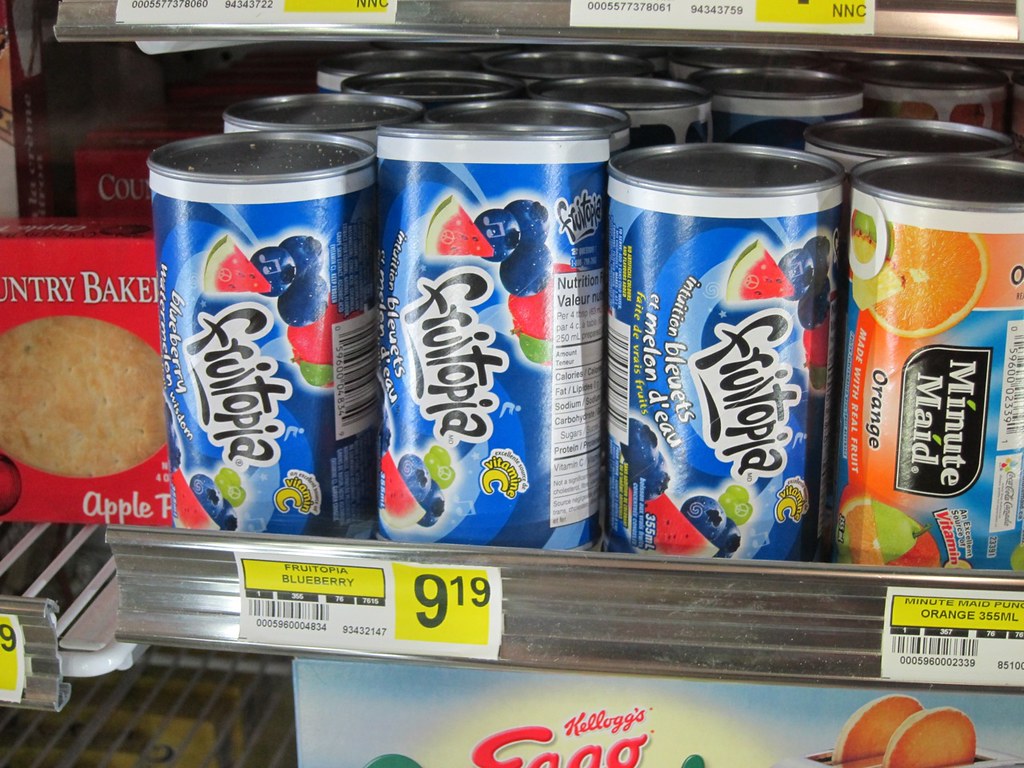Displayed on a neatly organized shelf within a supermarket, the scene features a silver display bracket prominently holding small pricing tags. Each tag is accented with vibrant yellow squares framing both the product name and price, complete with a small barcode for easy scanning. The shelf showcases an assortment of items starting with a single apple pastry on the left. This is followed by three rows of French fruit water cans labeled "Fruitopia Intuition Bluette et Melange d'eau," each priced at £9.19. To the right of these beverages, a lone can of Minute Maid orange juice stands out. The entire display is meticulously arranged, exuding the diversity and range of products available within the store.